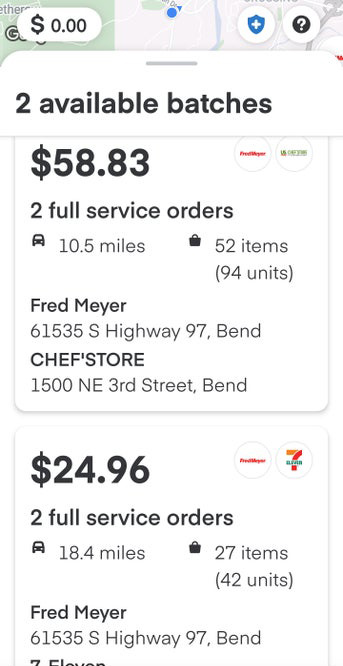Here is a cleaned-up and detailed caption for the image:

---

The image appears to be a screenshot from a food delivery application, possibly Uber Eats or a similar service. At the top section of the screen, there is a partial map with a white oval overlay, within which a dollar sign followed by "0.00" is displayed in black text. Below this, the screen indicates "2 available batches," suggesting options for delivery drivers to choose from.

The first available batch is highlighted and shows the following details:
- Payment: $58.83
- Type: Full-service orders
- Distance: 10.5 miles
- Items: 52 (94 units in parentheses)
- Store: Fred Meyer (a supermarket)

The second available batch is listed beneath with the following information:
- Payment: $24.96
- Further details are cut off in the screenshot but likely offer similar information regarding the type of order and distance.

Overall, the image provides a glimpse into the interface and options available to delivery drivers using this particular app.